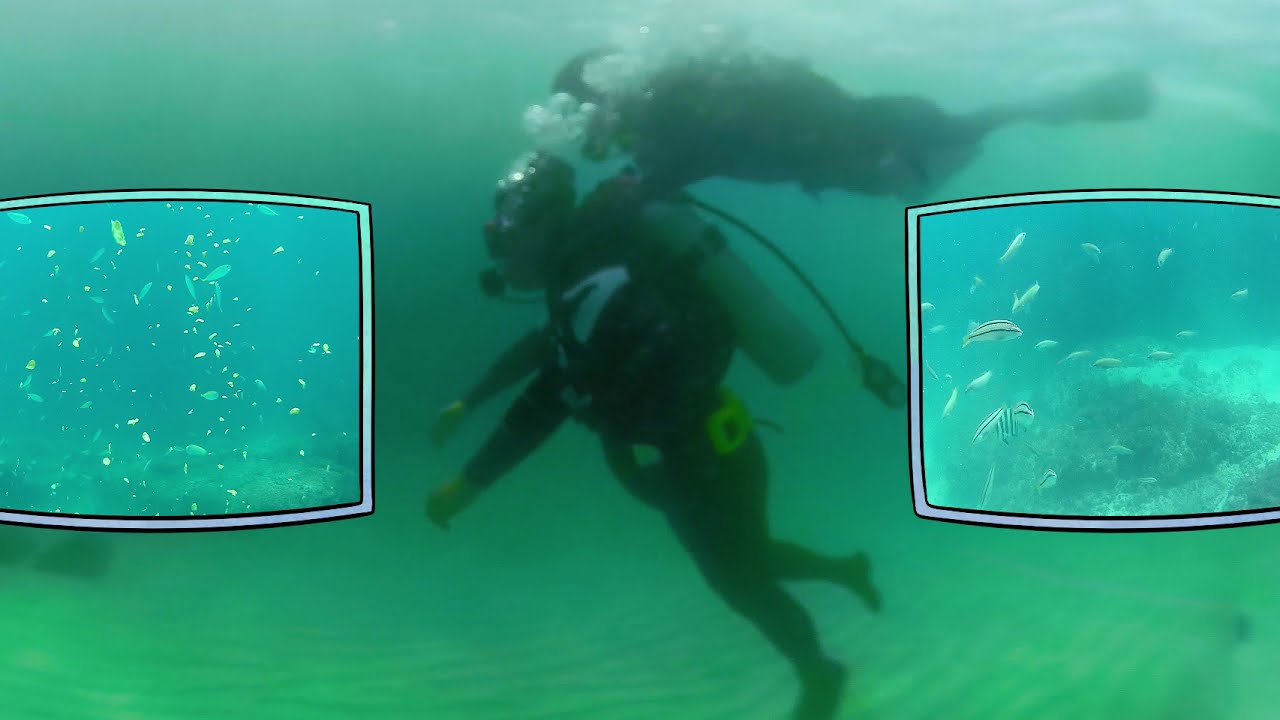The photograph captures an underwater scene featuring a scuba diver in full gear, including a wetsuit, mask, goggles, and an oxygen tank on his back, expelling bubbles from his mouthpiece. The diver, positioned near the murky, greenish-bottom of the sea, seems to be walking on sand dotted with stones. Above him, another diver floats horizontally, both moving towards the left side of the image. The surrounding water is a light, murky blue-green, enhancing the subaquatic atmosphere. Additionally, the image includes two square picture-in-picture inserts on either side, outlined in black. The left insert showcases a bright blue background with speckles, while the right features images of small fish amid a seabed, adding a touch of graphical contrast to the overall scene.